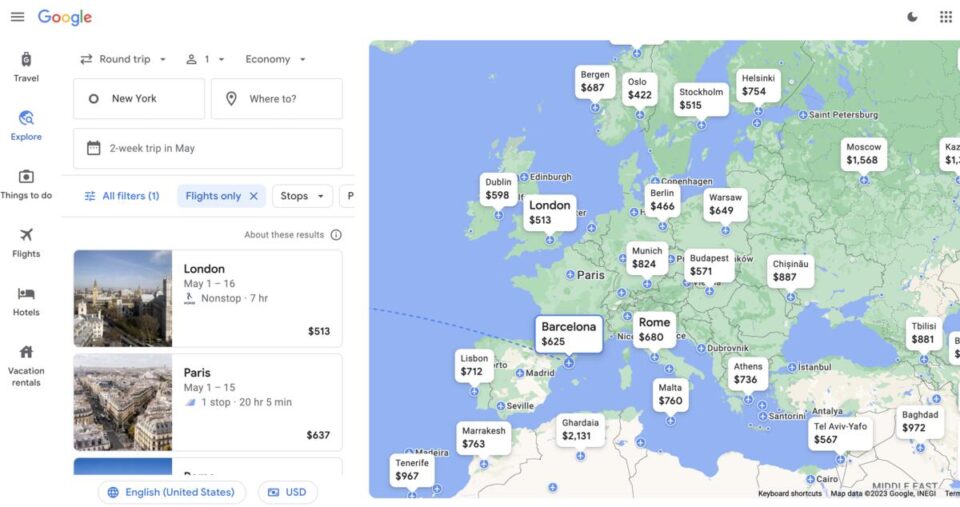Screenshot of a Google Explore page displayed on a desktop, laptop, or tablet. The interface features an extensive map predominantly showcasing Europe, parts of Russia, and the northern region of Africa. The map is dotted with tags denoting popular tourist destinations such as Barcelona, Rome, Munich, Budapest, London, Dublin, and Berlin, highlighting the non-stop round-trip prices available for these locations. 

On the left side, a graph appears to present a range of flight prices. The page offers numerous filtering options to refine search results, including preferences for round-trip or one-way travel, number of travelers, travel class (economy, business, etc.), departure and arrival locations, and trip duration.

Categories at the top of the page—such as 'Travel', 'Things to Do', 'Hotels', and 'Vacation Rentals'—provide further avenues for users to explore and plan their trips comprehensively.